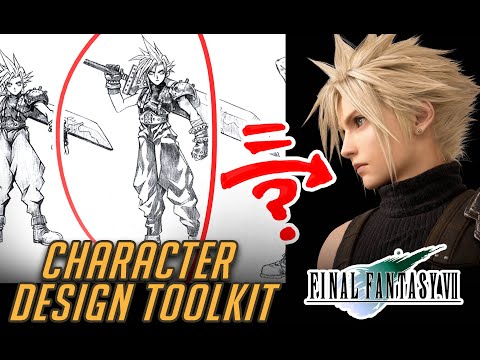This detailed image displays elements from the Final Fantasy series against a black background. Dominating the scene is a depiction of Cloud Strife, a central character from Final Fantasy VII. On the far right is a computer-animated rendering of Cloud, showing him in profile with his signature short, spiky blonde hair with tendrils falling around his face. He is dressed in a black turtleneck sweater with a black vest visible. The Final Fantasy VII logo, featuring a meteor in blue and teal, is clearly visible beneath the animated figure.

To the left of this rendering, there's a full-body black and white sketch of Cloud. The sketch showcases his iconic spiky hair, weightlifting belt, black pants, and a massive sword that extends down his back. He is also adorned with chains or metal bangles on his wrists and a single metal shoulder guard, highlighting his battle-ready appearance. The drawn figure of Cloud is surrounded by a red circle, with red arrows pointing towards the computer-generated character, accompanied by a red question mark underneath.

Above this sketch, in large yellow letters, the text "Character Design Toolkit" is prominently displayed. This text emphasizes the theme of character development and design within the Final Fantasy universe. Overall, the image brilliantly juxtaposes traditional sketch art with modern computer-generated imagery, encapsulating Cloud Strife's visual evolution in the iconic gaming series.